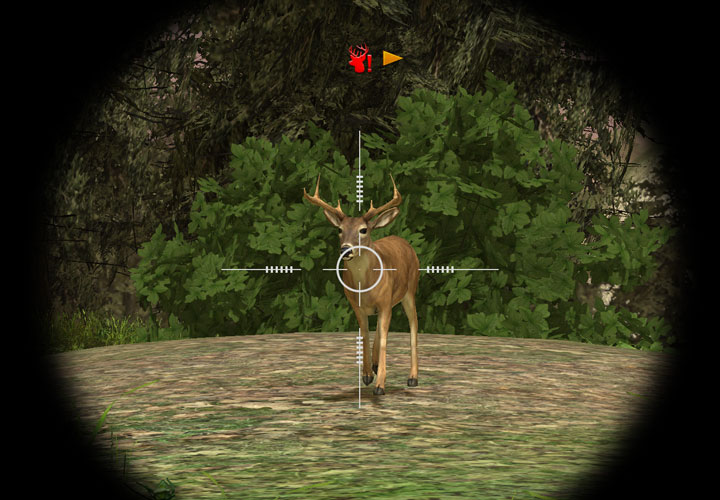The image appears to be a screenshot from a first-person shooter video game. In the center, the crosshairs of a rifle's scope are aimed precisely at a brown deer's jugular. Highlighted within the scope's white lens is the deer, which features small antlers resembling inverted stalactites and black hooves. The deer stands on a textured ground composed of varying shades of green, beige, and brown, representing a mix of grass, dirt, and soil. 

Surrounding the deer is a backdrop of green shrubs and trees with dark green leaves and brown branches. Adding to the immersive experience, the top of the image features a red deer head icon with an exclamation point, indicating the targeting of the animal, and beside it is a yellow forward arrow symbol and an orange play button, likely part of the game's interface.

Overall, the image's detailed graphics and smooth color transitions, combined with its artificial-looking greenery, indicate a sophisticated video game environment rather than a real-life scene.